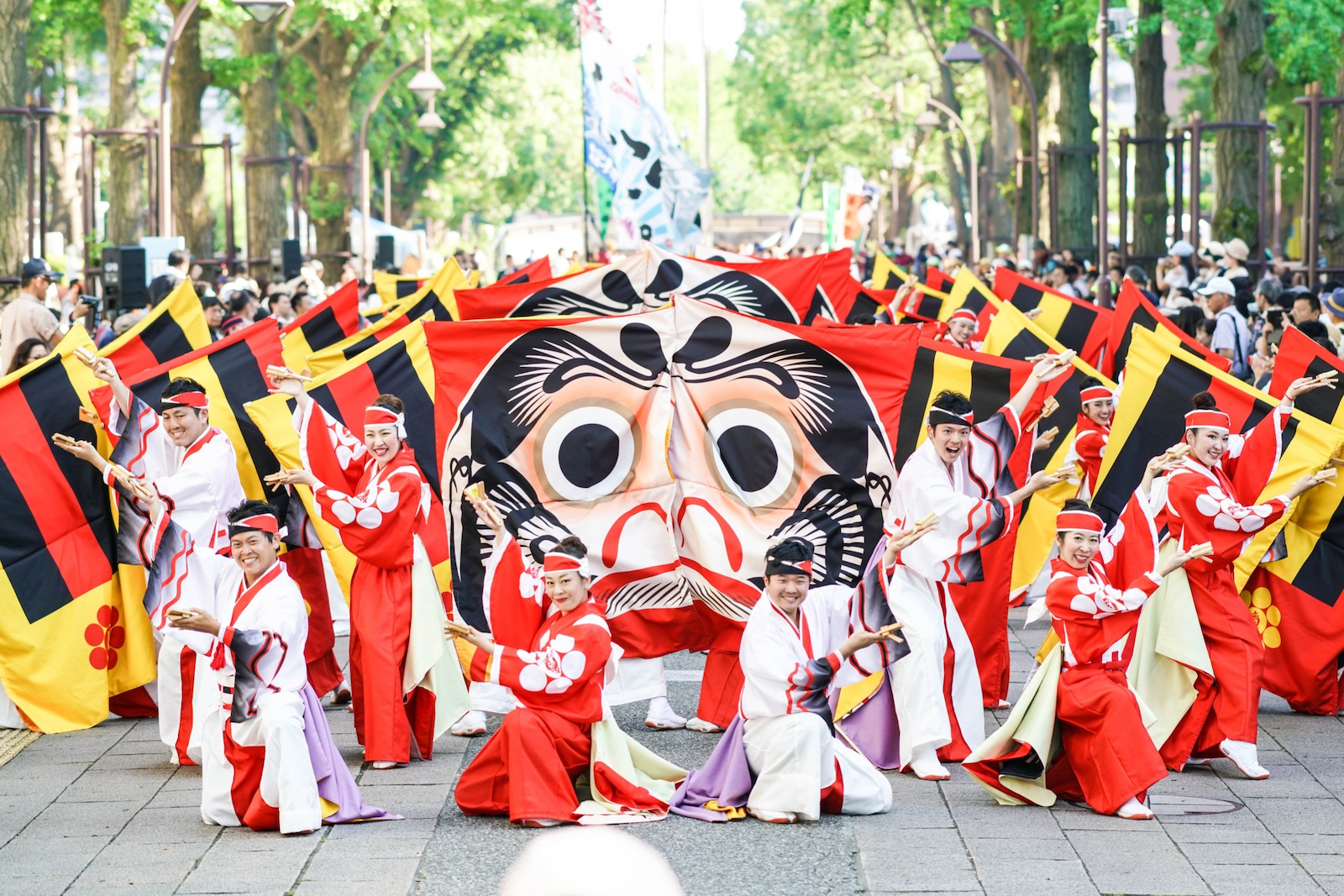The photograph captures a vibrant Japanese festival taking place outdoors during a sunny day. The central focus is a parade featuring elaborately dressed participants who appear to be performing a choreographed routine. The men are adorned in white robes with red trim, while the women are dressed in red robes with white floral designs on the sleeves. All participants wear headbands and display joyful expressions as they march down the gray, block-scored road.

In the background, various trees with brown bark and green leaves frame the image, with a bright piece of sky visible at the top center. Among the flags and banners being carried, a prominent white, black, and greenish-blue flag stands tall above the crowd, along with yellow flags featuring red and black stripes in the center top section of the image. Additionally, spectators can be seen on either side of the street, capturing the lively event with their cameras. The scene is set against a backdrop of white trees, adding to the festive atmosphere.